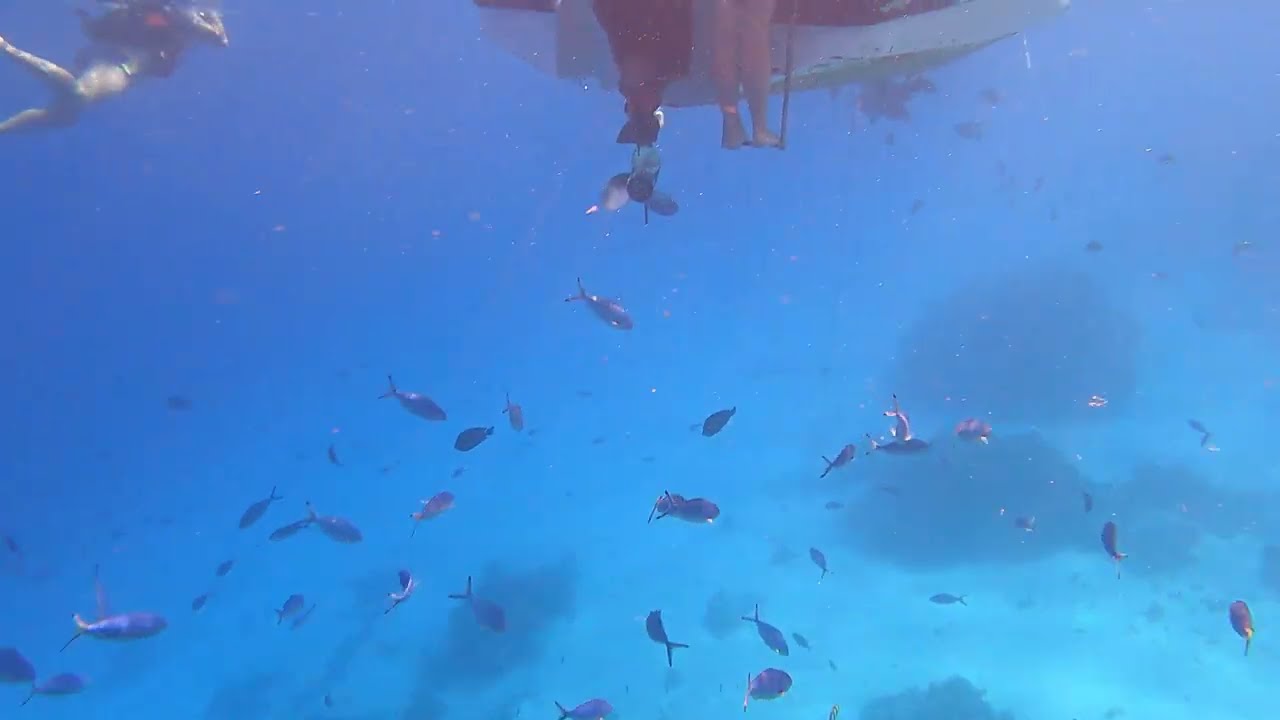The underwater photograph showcases a clear aquatic scene teeming with details. At the top of the image, three people create a dynamic composition. To the top left, a woman wearing bikini bottoms and some sort of vest is seen swimming. In the center top, the bottom of a boat with a visible propeller and partial submersion creates a striking centerpiece. Adjacent to this is a pair of legs belonging to a person standing on a ladder attached to the stern of the boat; the person on the left is clad entirely in black up to the visible upper leg, while the person on the right is barefoot with a distinctive pink strap around their left leg. Below this human activity, the scene flourishes with a large school of grayish fish, likely numbering in the dozens, swimming near the sandy ocean floor dotted with large rocks. The overall clarity of the water reveals a vibrant underwater environment, hinting at an offshore sea location.